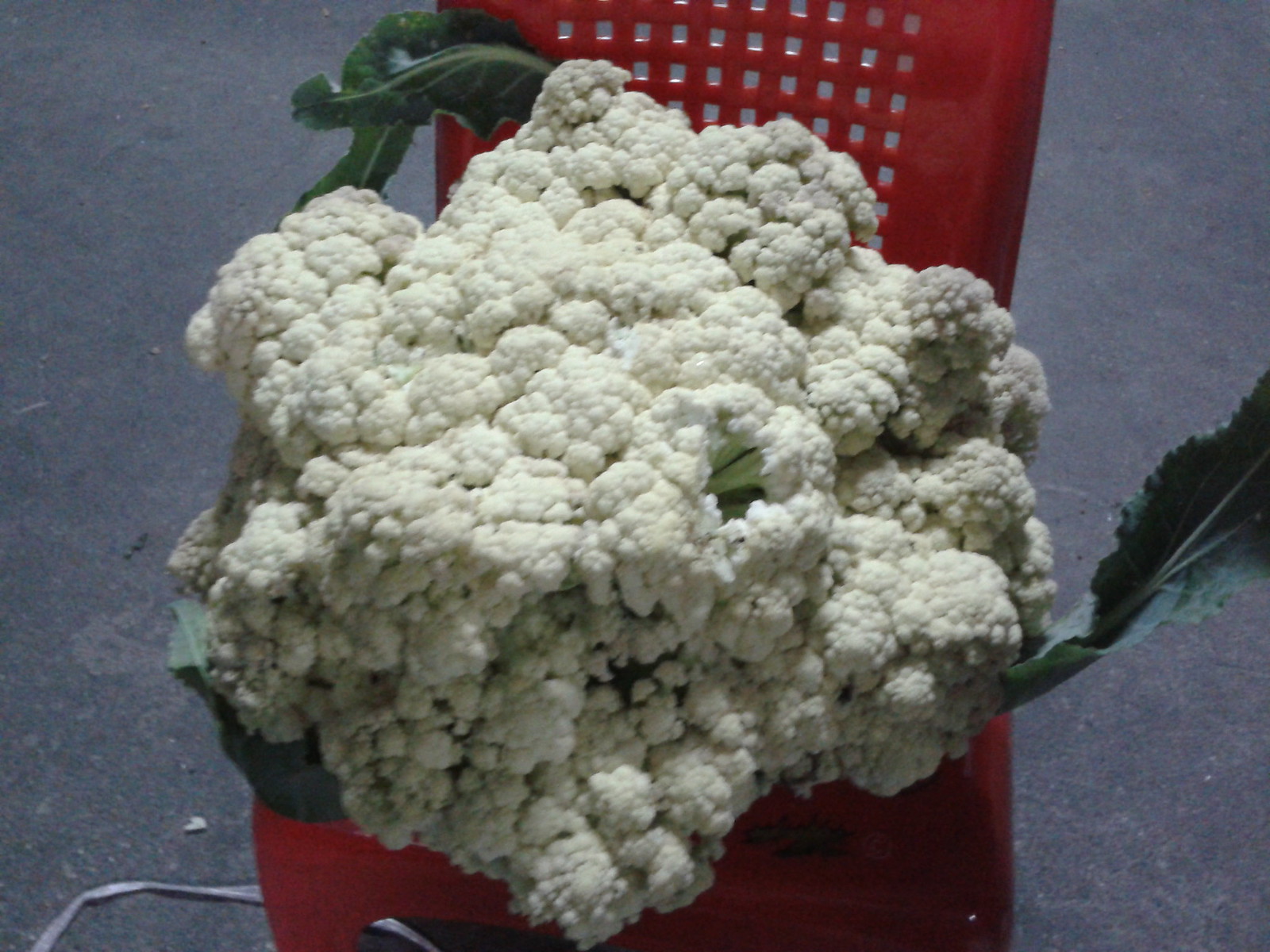The photograph depicts a whole, white, and fluffy cauliflower sitting in a red plastic container, which resembles a red plastic chair with decorative holes on the back. The voluminous cauliflower, about the size of a large bundle and possibly resembling marshmallows or popcorn, showcases its intact form with no chunks removed. Nestled among the vegetable's textured surface are three large, dark green leaves that protrude visibly. The container sits on a gray base, likely a gray asphalt floor or a short gray carpet, and the overall setting appears somewhat cloudy with no strong lighting visible.